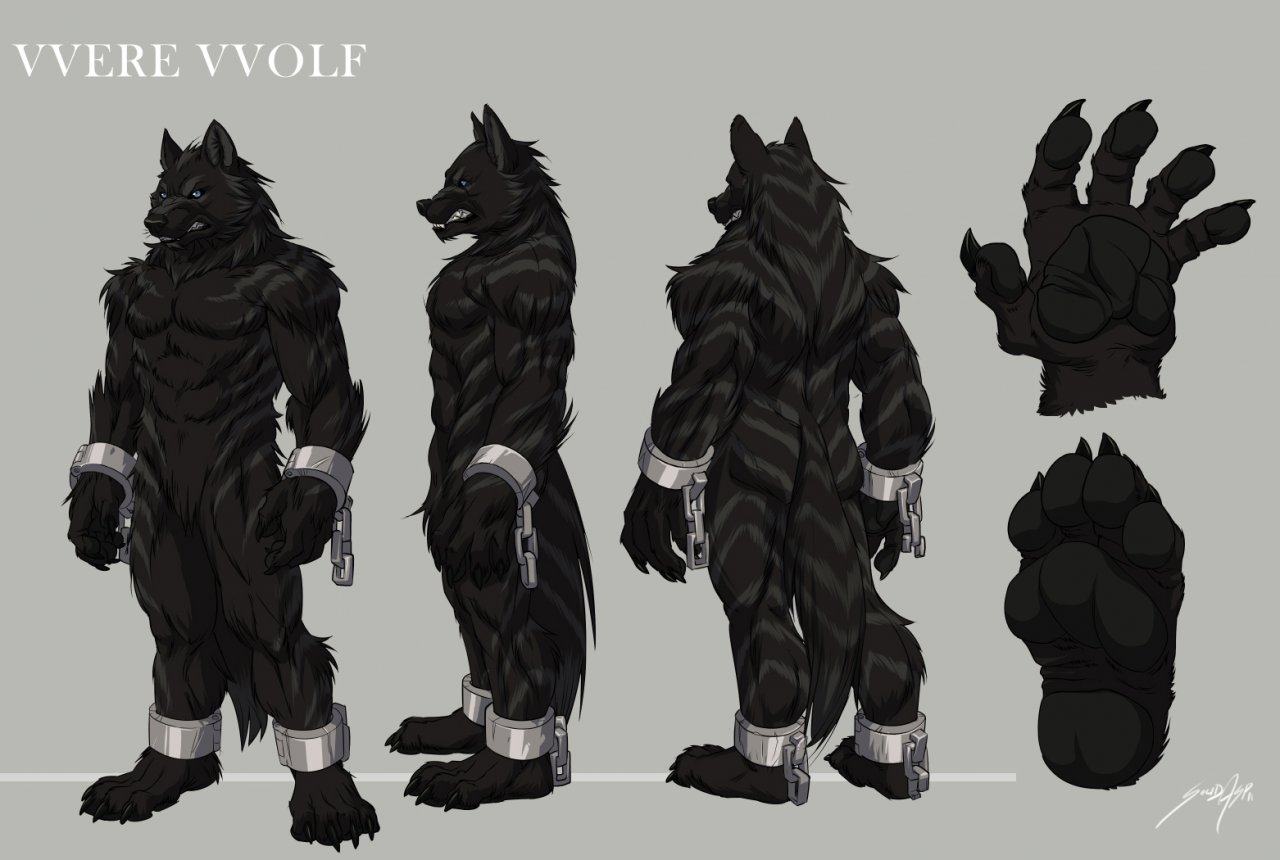The image features an artistic rendition of a black-furred werewolf standing upright in four distinct poses against a light gray background. In the upper left corner, "VVERE VVOLF" is written in white letters. The werewolf has muscular features, pointy ears, a dog-like snout, striking blue eyes, and bared teeth. It is adorned with silver shackles on its wrists and ankles, with broken chains hanging from them. The werewolf's fur includes subtle gray striping, adding to its menacing appearance. The first pose shows the werewolf looking diagonally forward, the second provides a side profile, the third depicts its back, and the fourth section includes close-ups of its hand with sharp claws and its clawed foot. The extreme detail and dynamic poses emphasize its readiness for battle.